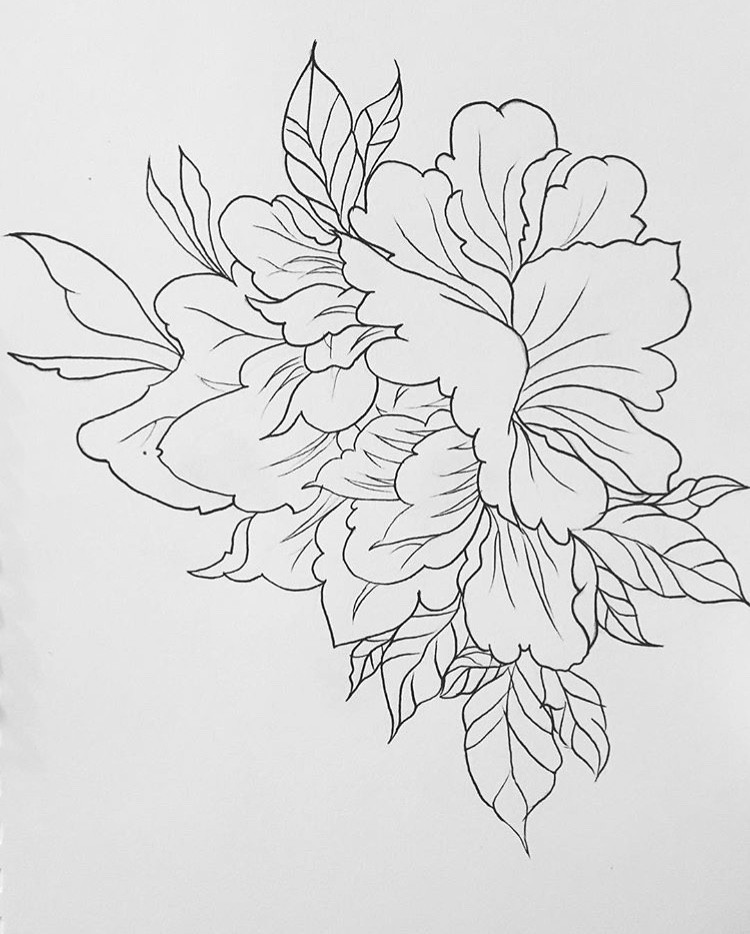In this intricate sketch, a harmonious arrangement of flowers and leaves unfolds, starting from the bottom right corner and extending towards the center and upper portions of the image. The composition begins with two distinct leaves in the lower right, transitioning into a cluster of additional leaves on the left. Ascending from this base, a prominent flower structure emerges on the left-hand side, dominating the sketch with its size and detail. Around this central bloom, smaller floral elements and leaf shapes extend outward, particularly towards the upper left. The entire sketch is set against a subtle, light gray background that spans the entire canvas, providing a gentle contrast that highlights the detailed and interconnected botanical elements within the scene.